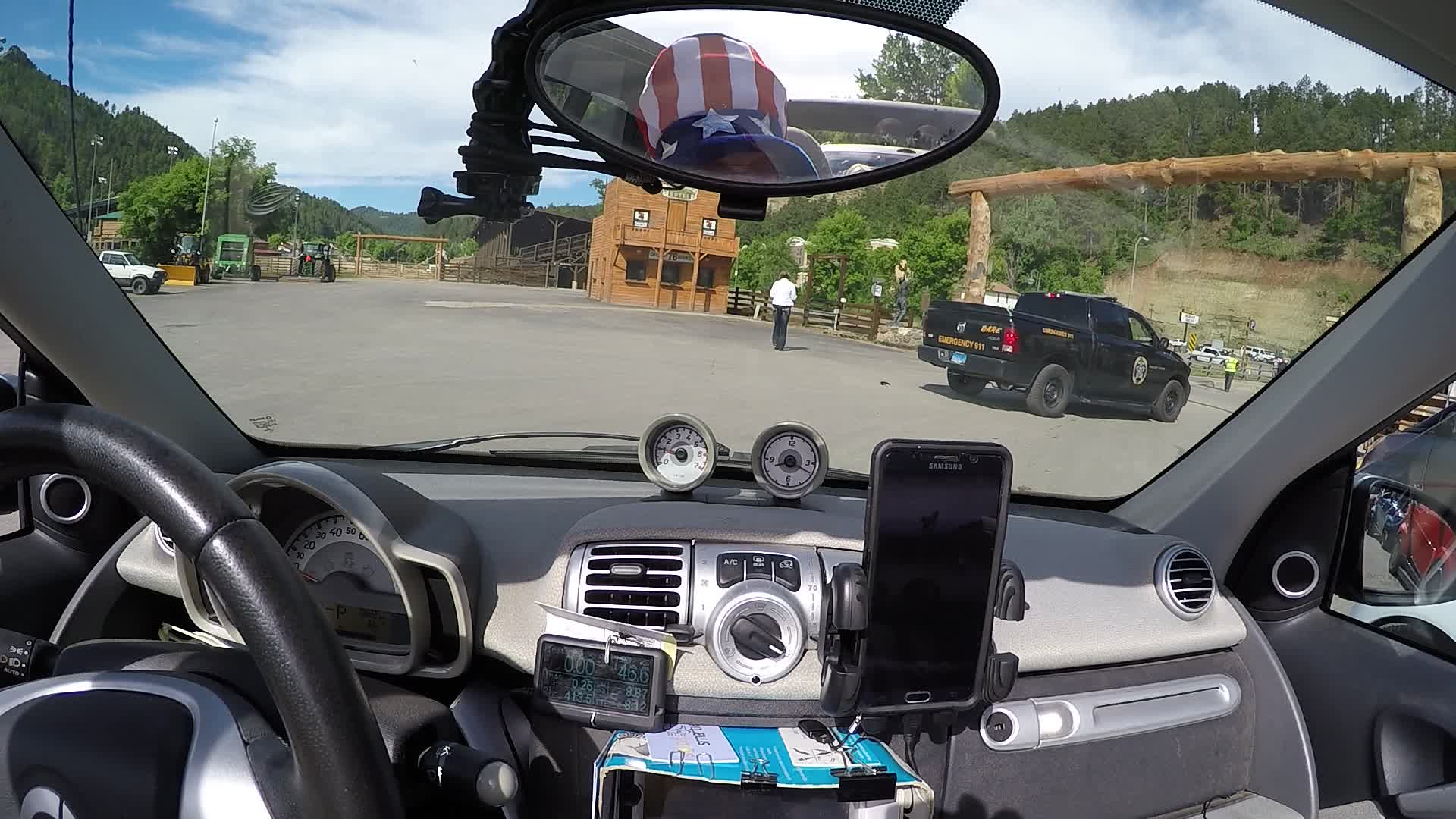The photograph, taken in landscape format and in color, captures the interior of a very small car from the driver's seat, presenting a detailed view of the dashboard and windshield scenery. The steering wheel is on the left side, indicating a left-hand drive vehicle. The interior is a blend of silver and black components, featuring a display panel and several added circular gauges on the top of the dashboard. A smartphone, held in a holder, is attached to the center console, surrounded by papers and cards clamped in an unusual manner. The prominently visible rear-view mirror is circular, enhancing the distinct European design of the compact car, although the style inside is very American. Reflected in the mirror is an individual, presumably the photographer, wearing or capturing an image of someone wearing an Uncle Sam hat adorned with red, white, and blue stripes. 

Through the windshield, the backdrop reveals a picturesque day with a bright blue sky and fluffy white clouds. In the foreground outside, a black pickup truck is parked, and beyond it, lush greenery with mountains and trees hints at a park-like setting. The vista is dominated by an Old West theme park entrance, complete with rustic storefronts evocative of a bygone era. The scenes inside and outside the car merge into a single narrative of nostalgia and exploration, framed by the quaint yet adventurous spirit of the theme park.